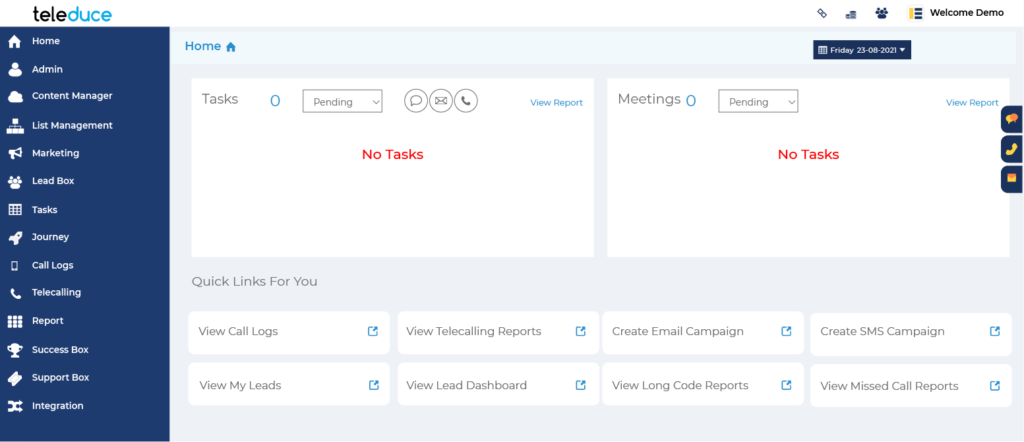The image depicts the home page of TELEDUCE, a web application interface. The logo "TELEDUCE" is prominently displayed at the top, with "TELE" in black and "DUCE" in a bright sky blue color. The left-hand side of the screen features a vertical navigation menu with clickable sections, each encapsulated in a blue box with white text. The available categories include Home, Admin, Content Manager, List Management, Marketing, Lead Box, Task, Journey, Call Logs, Telecalling Reports, Success Box, Support Box, and Integration. Each category is accompanied by a distinct icon.

At the center of the screen is the main display area showing the home section, marked by a small house icon also in sky blue. The current date, Friday, August 23rd, 2021, is displayed prominently to the right of the home icon. Below the date, two large rectangular status boxes indicate "Tasks" and "Meetings," both showing zero with "No tasks" and "No meetings" in red text.

The bottom of the interface contains a row of quick links for essential actions, each housed in small white boxes. These quick links include options such as View Call Logs, View My Leads, View Telecalling Reports, View Lead Dashboard, Create Email Campaign, View Long Code Reports, Create SMS Campaign, and View Missed Call Reports.